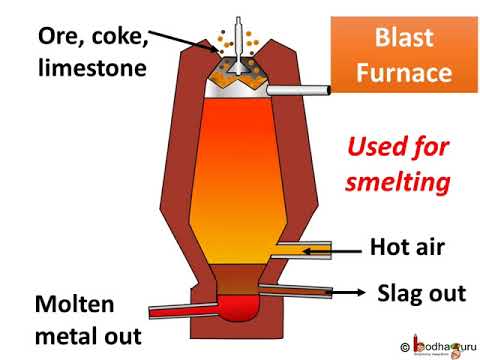The illustrated image portrays a detailed diagram of a blast furnace, prominently labeled as such. The furnace itself is shaped like an upside-down soda bottle, enveloped in a thick maroon lining. It features a vertical gradient of colors: transitioning from orange at the top, through yellow and brown, to a deep red at the bottom. At the apex of the diagram, there's an aperture labeled for the entry of ore, coke, and limestone. The furnace's functioning is described with notes indicating that it is used for smelting. Detailed labels in the diagram point out the induction of hot air at the bottom, with dedicated exits for slag and molten metal. Additionally, the bottom right corner of the image features the copyright marking "B-O-D-H-A-G-U-R-U."